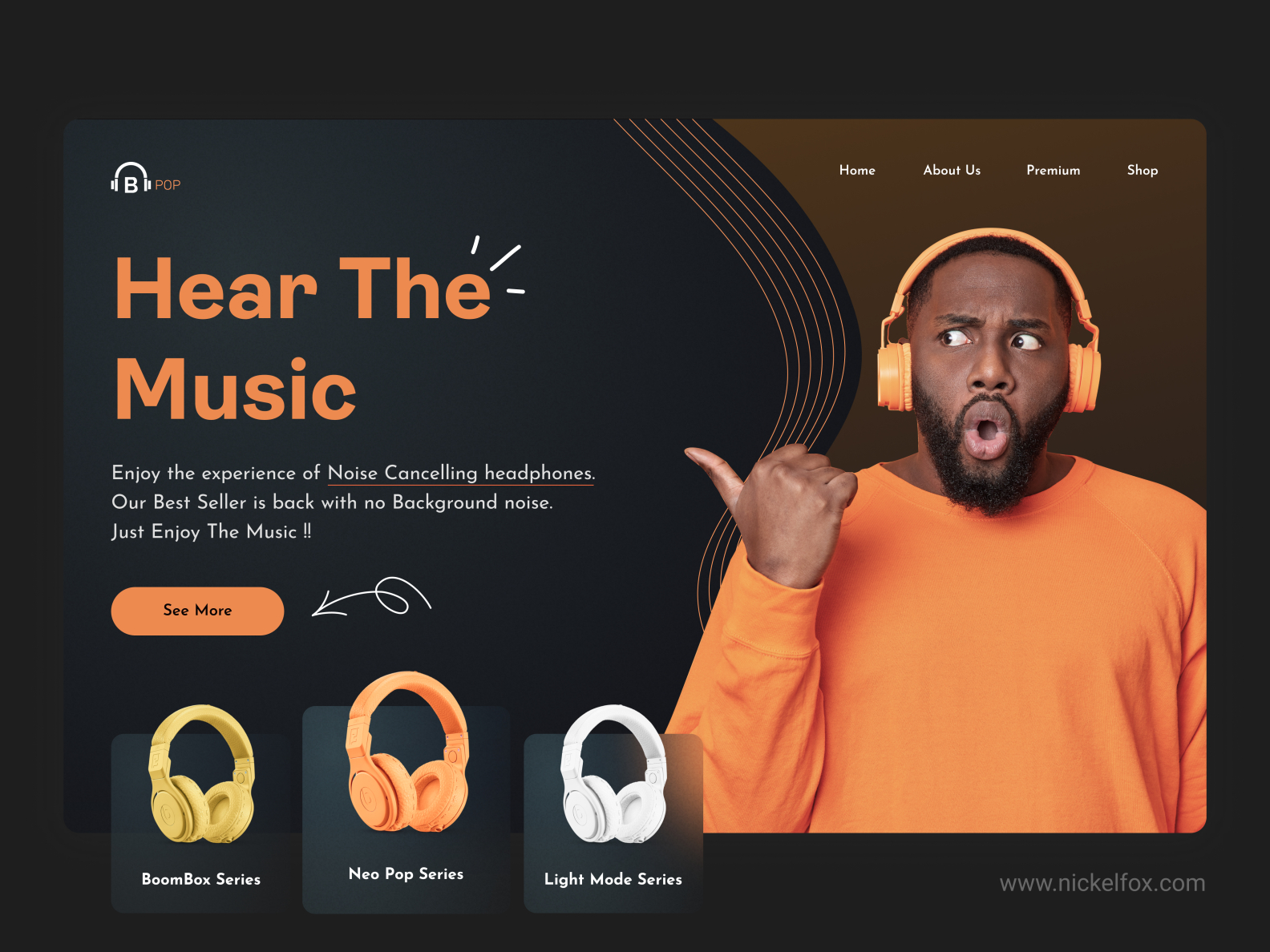The image is a vibrant and engaging screen grab, potentially for an advertisement or splash screen for a website, featuring the URL www.nickelfox.com prominently displayed in the bottom left corner. Dominating the right half of the screen is a man adorned in an orange shirt and matching orange headphones, exuding a sense of energy and style. 

On the left side, the captivating text "Hear the Music" is displayed in bold orange, harmonizing with the man's attire and headphones. Notably, the 'E' in "the" features three dynamic lines emanating from it, symbolizing sound waves or volume indicators, adding a creative visual touch.

Beneath this, in contrasting white text, is a compelling tagline: "Enjoy the experience of noise-cancelling headphones, our bestsellers are back with no background noise. Just enjoy the music." This message underscores the premium audio experience offered by the featured products.

An eye-catching orange button labeled "See More" invites viewers to explore further. Below this call-to-action are three showcased over-the-ear headphones: 
1. The Boombox Series in vibrant yellow,
2. The Neeko Pop Series in striking orange,
3. The Light Mode Series in sleek white.

Each product is clearly named and distinctively colored, emphasizing the diversity and appeal of the headphone range on offer.